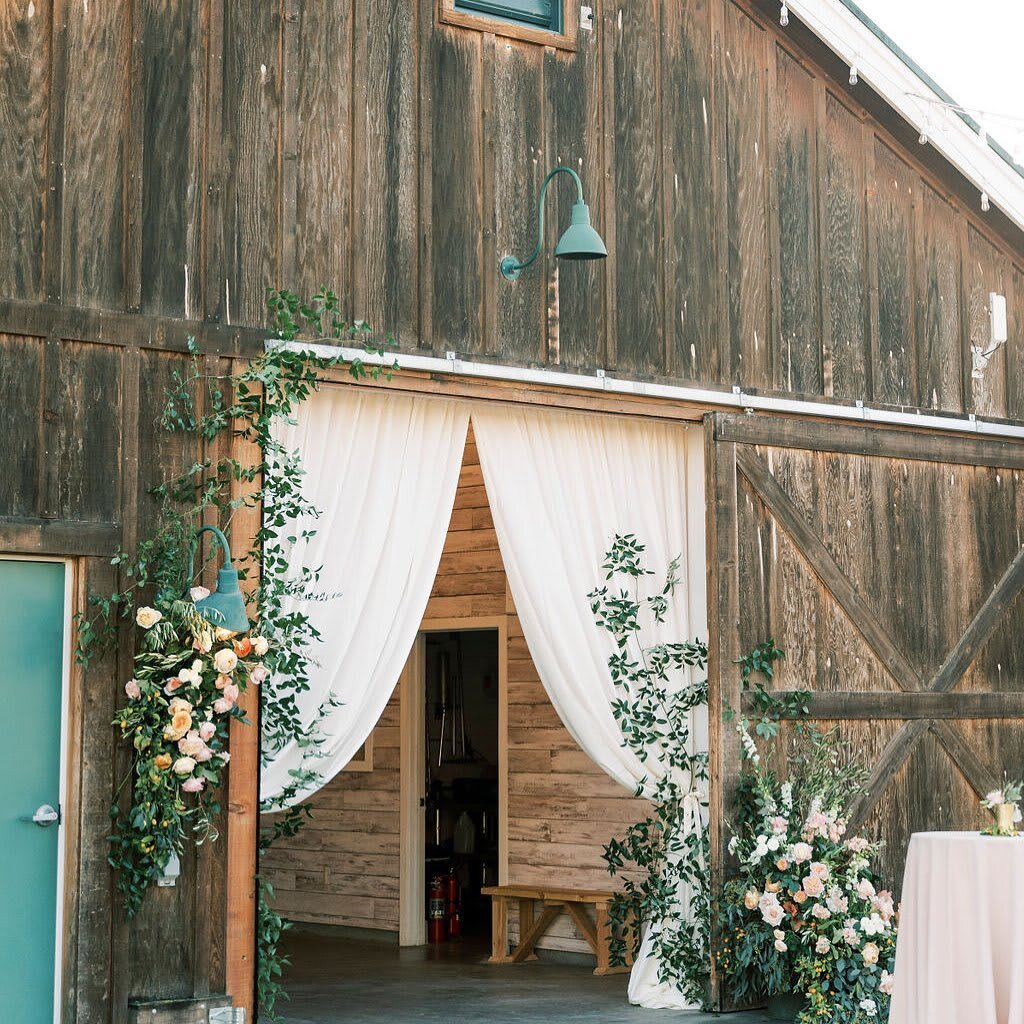This outdoor image showcases a large, weathered wooden building that evokes the charm of an old barn or a rustic cabin. The structure's facade, made of brown unpainted wood, occupies most of the frame, contrasted by a striking green door on the far left. Central to the composition is an inviting entrance, framed by white curtains that are drawn open, revealing a cozy interior. Above this opening, a distinctive green light fixture extends outward and then points directly downward, ready to cast its illumination. Inside, a small wooden bench sits adjacent to another doorway, where glimpses of equipment, including fire extinguishers, can be seen.

Around this central entrance, the scene is softened by clusters of green plants and vividly pink roses, adding a touch of natural beauty to the rustic setting. Additionally, a round table adorned with a white tablecloth and a central arrangement can be spotted towards the bottom right of the image, hinting at the warmth and liveliness within this serene outdoor capture. The bright daylight filtering through the scene further emphasizes the building's well-worn character and the vibrant life surrounding it.